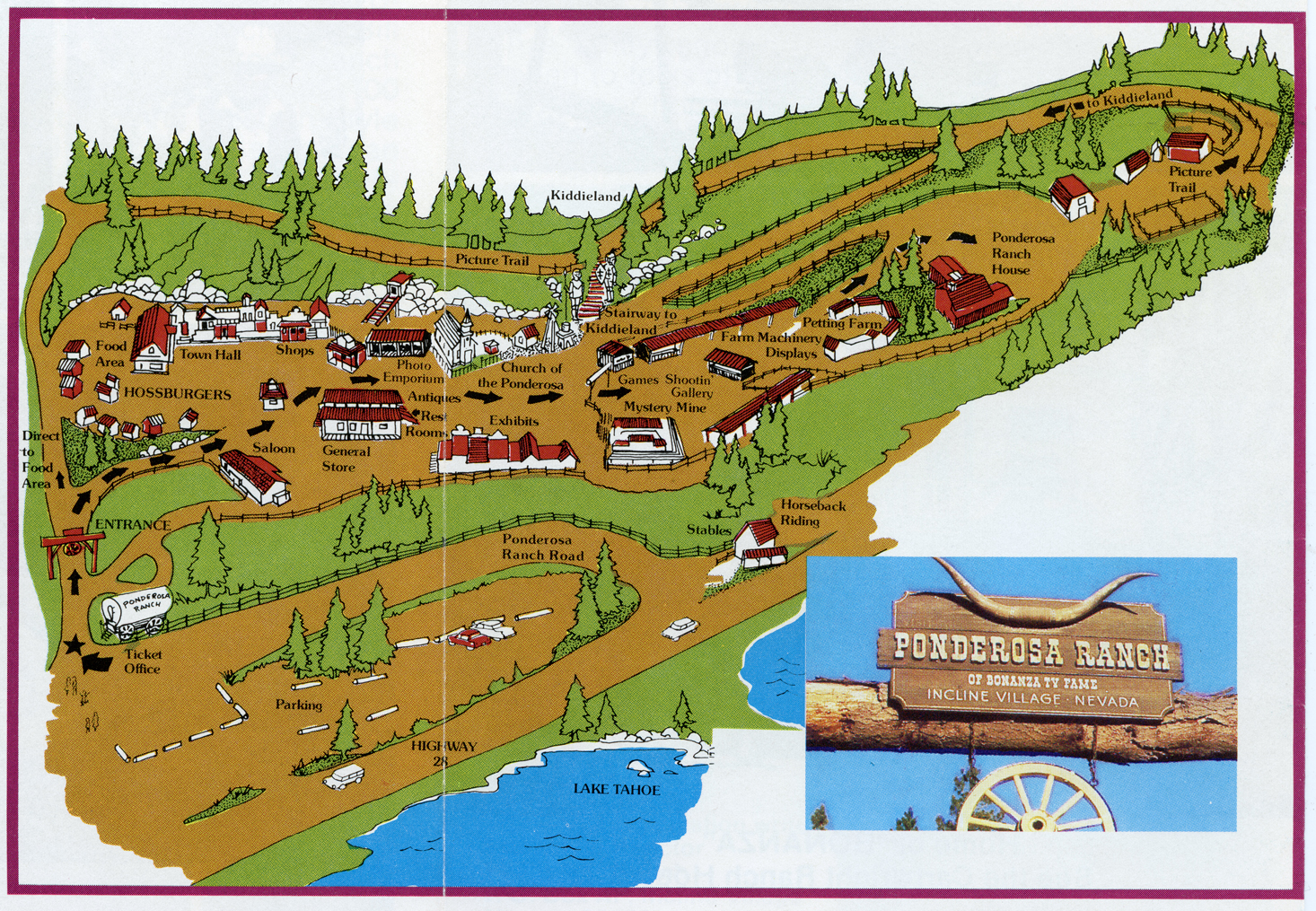This detailed image showcases an animated map of the Ponderosa Ranch, highlighted by an authentic photograph of a brown wooden sign with bull horns and a wagon wheel, located in the bottom right corner. The sign prominently reads "Ponderosa Ranch of Bonanza, TY fame. Incline Village, Nevada" in white font. The map, framed by a solid fuchsia border with the illustration centered in a white space, depicts intricate details of the ranch. The green areas signify grass, punctuated by numerous illustrated pine trees. A blue section labeled "Lake Tahoe" is situated at the bottom of the map. Moving upwards from the lake, areas of brown land are interspersed with white buildings characterized by dark red roofs. Each building, along with the main roads and areas, carries small black text labels. The map outlines various features including farmland or a village with visible dirt roads, parking spaces, and numerous labeled buildings such as a food area, town hall, shops, general store, and saloon. Notably, a large trail leads into a section marked as "kiddy land." The field appears expansive, dotted with parked cars, adding to the lively depiction of Ponderosa Ranch.